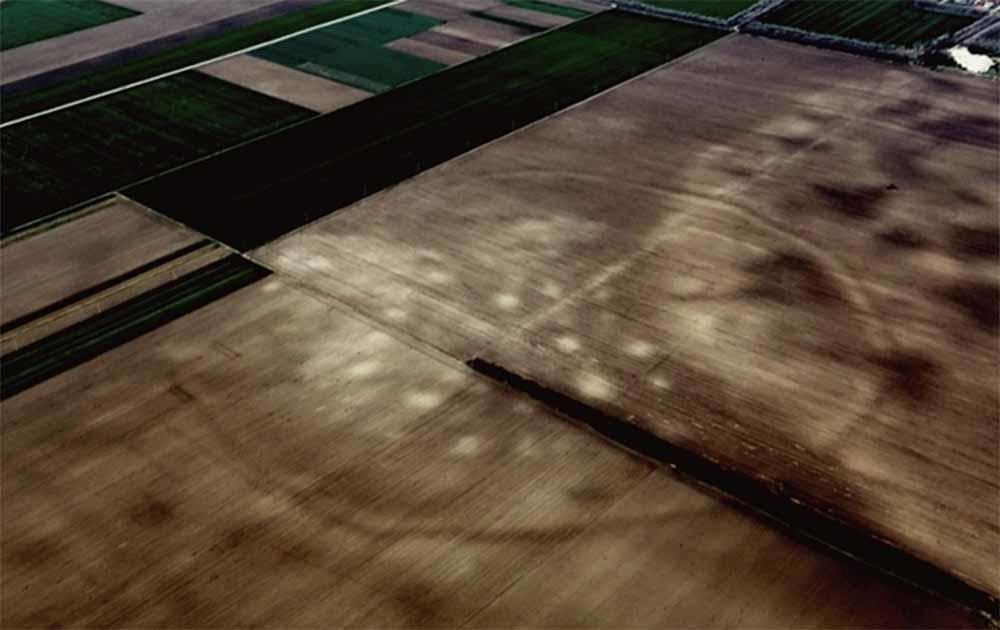This image is a rectangular digital photograph, approximately 6 inches wide and 3 inches high. It captures an aerial view of a farmland scene, but the lighting conditions make it quite dark, especially in the upper left and right corners, as well as along the right-hand side, which is heavily shadowed. The photograph features several rectangular and diagonal patches of varying shades of green and brown, indicating different types of fields and stages of crop growth.

In the upper left quadrant of the image, there are diagonal rectangles in dark green and light tan, which likely represent different vegetable farmlands. These patterns continue until about two-thirds of the way across the top. Below these, towards the right, are two sections of light brown, which could be interpreted as planks of wood or tilled soil, perhaps demarcating different farms.

In the upper right portion, additional green farmlands and some buildings are visible. The image is characterized by a mix of fields in shades of dark green, light green, and brown, creating a patchwork effect typical of farmland. Shadows, perhaps from trees, add to the complexity of the landscape. Despite the overall darkness and possibly blurred quality of the photo, it distinctly depicts a cultivated area with various crops.